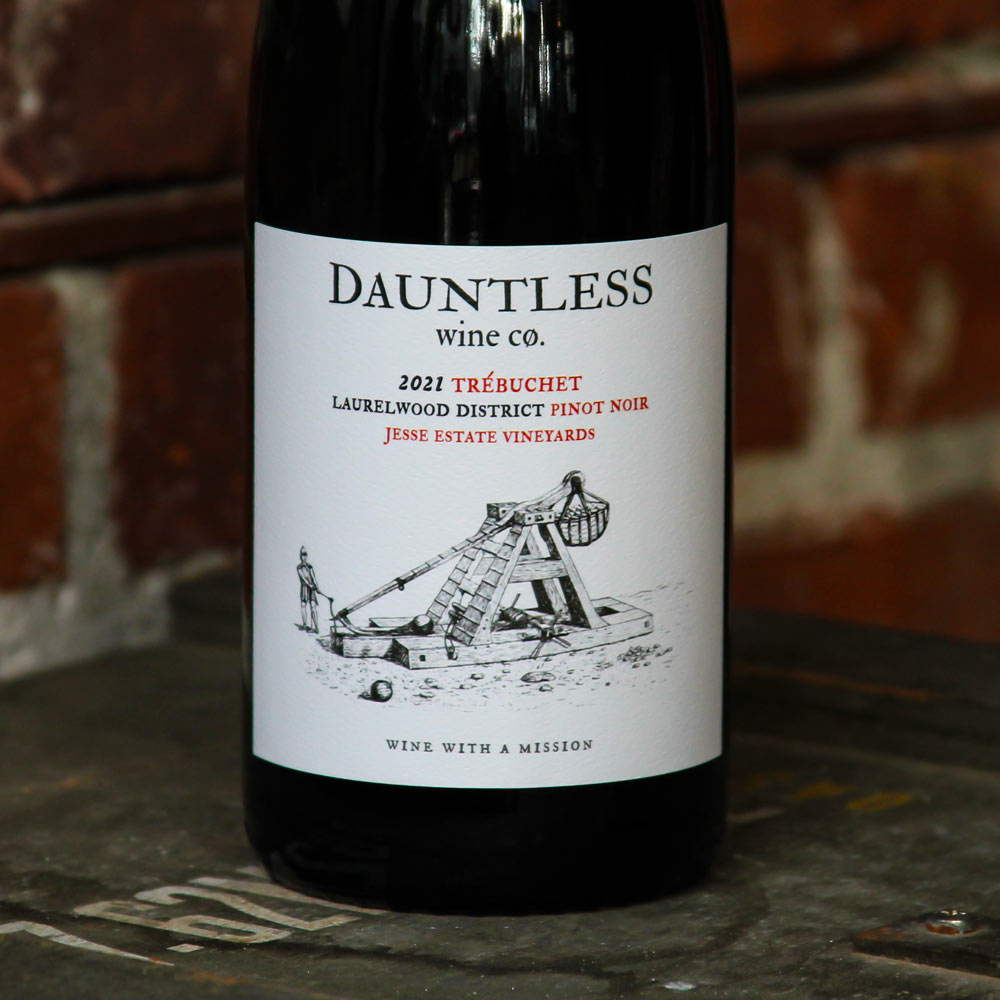This professionally taken photograph showcases a close-up of a premium bottle of wine, with a strong focus on the intricately designed label. The bottle, which is partially captured, sits on a textured gray surface that displays a series of numbers and hexagons, suggesting a metallic material. Behind the bottle, a red and white brick wall provides a subtly blurred backdrop, enhancing the clarity and prominence of the label.

The label itself reads "Dauntless Wine Company" in bold black lettering, followed by the year "2021" in smaller black text. The centerpiece is the word "Trebuchet," elegantly depicted in red with an accent on the 'e.' Below this, "Laurelwood District" and "Pinot Noir" are positioned in black and red text respectively, followed by the smaller black text identifying "Jesse Estate Vineyards." At the bottom of the label, the company's slogan "Wine with a Mission" is clearly displayed.

An intricately detailed graphic of a medieval trebuchet, a historical catapult-like device, is also featured on the label, adding an element of intrigue and craftsmanship. The image suggests a careful blend of tradition and quality, implying that this might be a high-end brand of wine, potentially part of a promotional campaign or a professional product feature.